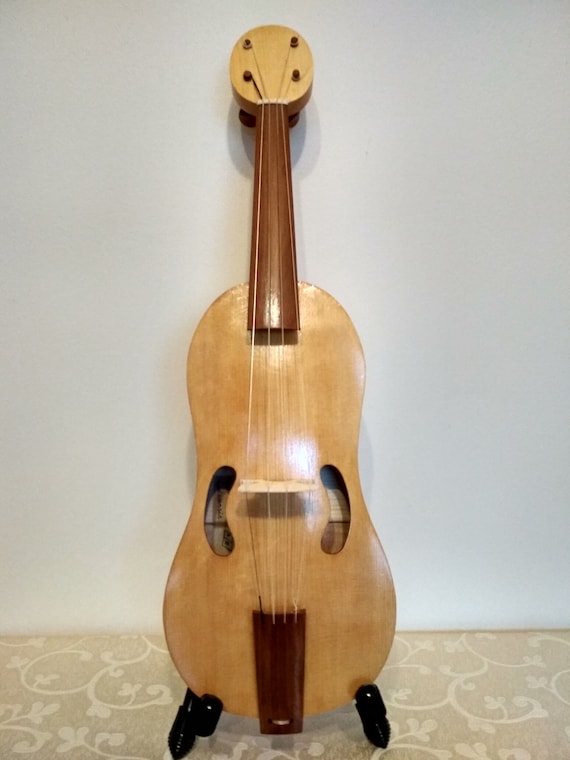This color photograph features a stringed instrument, prominently upright on a stand with shiny black feet, which could be plastic or metal. The floor it rests on is brown and adorned with white stylized flowers, contrasting against a plain gray wall in the background. The instrument itself resembles an old violin, with a body crafted from light, glossy tan wood. The four white strings stretch from the top to the bottom, anchored by a light wood bridge in the middle. 

Its body showcases a curvy silhouette, narrowing at the center and expanding towards the top and bottom, where it features two curved sound holes flanking the strings. The instrument has a dark brown neck that extends to a headstock of matching light wood, rounded at the top. The headstock is equipped with two tuning pegs for adjusting the strings. The entire setup suggests a casual, possibly unprofessional product listing, perhaps by someone looking to clear out space at home. This staging gives it a charming, homey feel, capturing the essence of a cherished musical piece ready for a new owner.